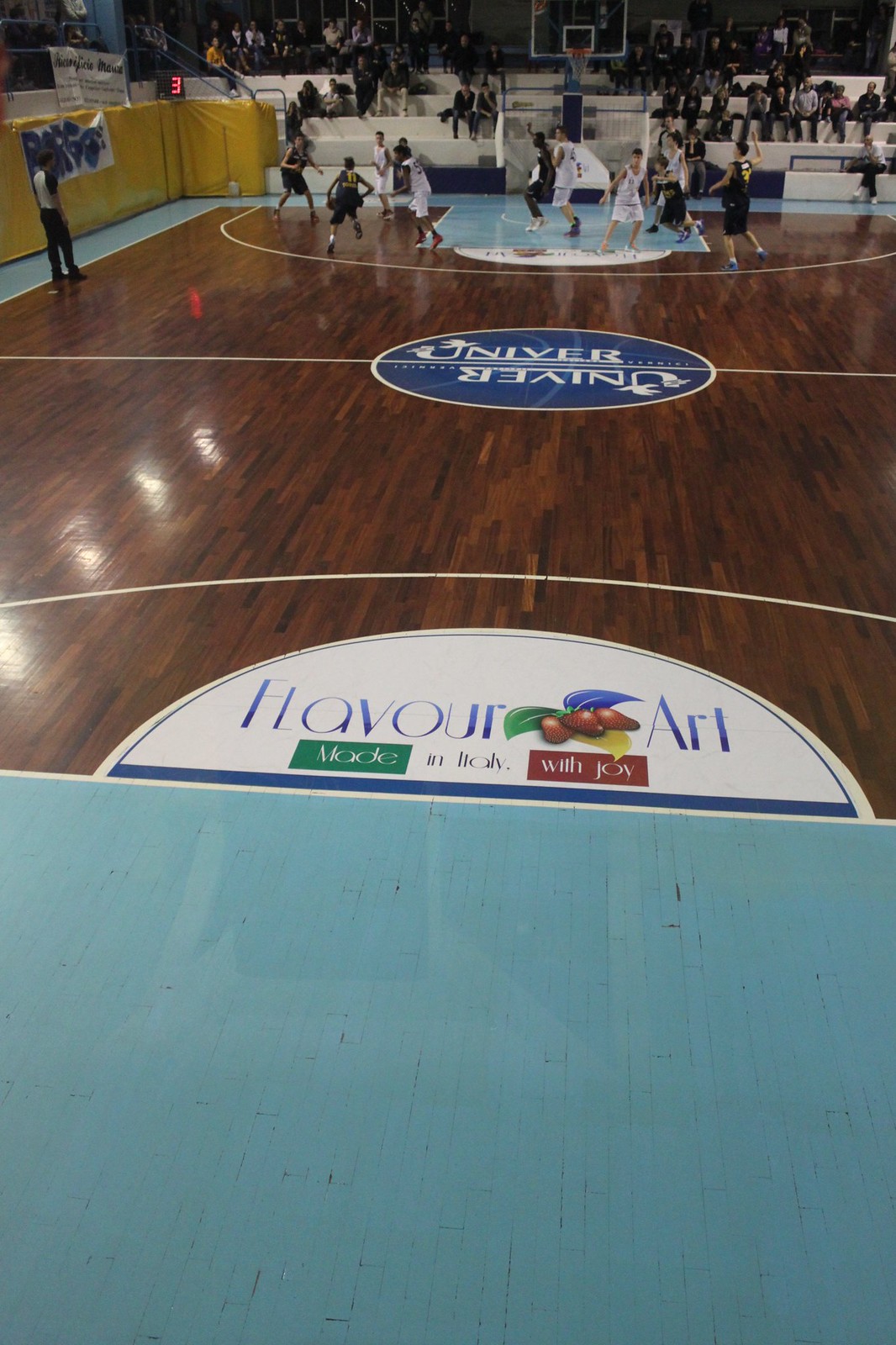This rectangular image captures a dynamic basketball game from an elevated perspective slightly behind the near basket. The photograph showcases the entire length of the court, with the action concentrated at the far end where players in contrasting uniforms—white with black lettering and black with yellow lettering—engage fervently. The court itself is predominantly dark brown hardwood, interspersed with a light blue painted area near the hoop and a central dark blue circle emblazoned with “UNIVER” in white text. Adjacent to the blue painted area is a semi-circular logo featuring “FLAVOR ART” flanked by a trio of colorful leaves and individual strawberries, alongside the text “Made in Italy with joy,” accented by red and green boxes. Spectators fill the white bleachers that ascend behind the distant players, adding a vibrant backdrop to the game. A wall on the left, padded and yellow, also features a white sign with blue text. The presence of referees and the vivid contrasts of the court components add further life to this energetic sports scene.